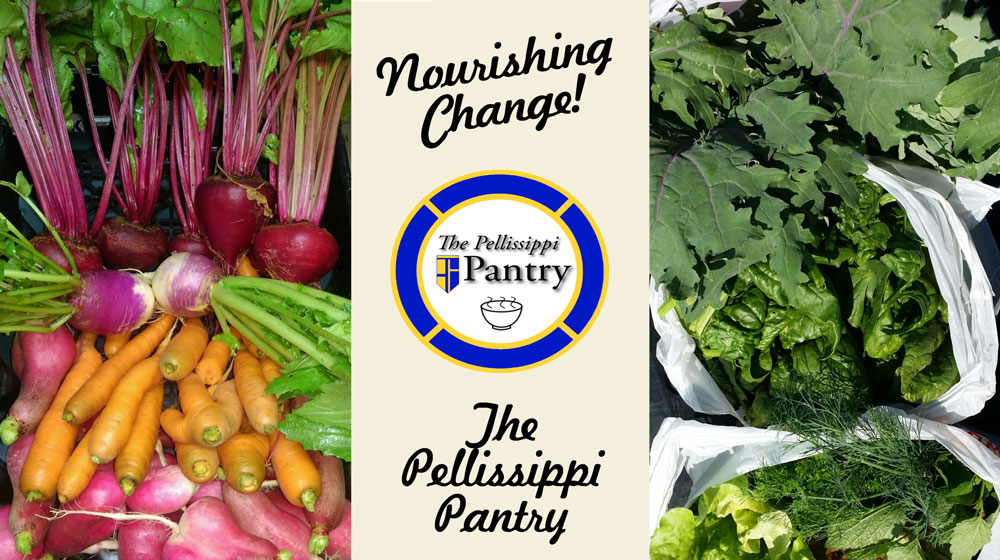The image is a visually striking advertisement for the Pellissippi Pantry, focusing on fresh produce and greens. On the left side, there's an enticing assortment of colorful vegetables including radishes, carrots, and various leafy greens, vibrant with reds, oranges, and greens. The right side contrasts this with neatly packaged greens displayed in white bags. Centered between these two sections is a white panel featuring black script text that reads "Nourishing Change." Above this text, there is a distinctive blue-bordered circle containing the words "The Pellissippi Pantry," accompanied by a logo resembling a blue open door on a yellow background. This visually engaging image appears to be aimed at promoting healthy eating through the Pellissippi Pantry's offerings, possibly showcased at a farmer's market.